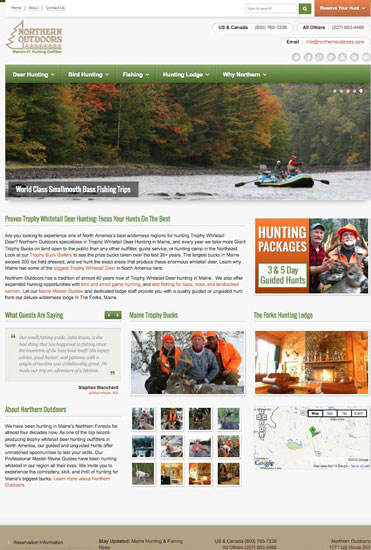The image depicts a screenshot of a web page for Northern Outdoors, an outdoor adventure company catering to enthusiasts in the U.S. and Canada. At the top of the page, there is a search bar featuring a green magnifying glass and a small, unreadable orange rectangle button. The site’s name, "Northern Outdoors," is prominently displayed in brown text alongside a pine tree logo. The page header includes contact information such as an 800 phone number and tabs for "All Orders" and email options. Social media icons for Twitter, Facebook, and Instagram are also present.

Below the header, there is a navigation bar with a green background containing dropdown menus for "Deer Hunting," "Bird Hunting," "Fishing," "Hunting Lodge," and "Why Northern."

The main section features a photograph of an autumn landscape, with vibrant fall foliage in shades of red, yellow, and green. In the foreground, two individuals are in a boat on a river, seemingly engaged in fishing. Overlaid text promotes "world class smallmouth bass fishing trips" and offers hunting packages for three and five days, including guided hunts. The page also includes a photo of three men proudly holding a deer, highlighting successful hunting expeditions.